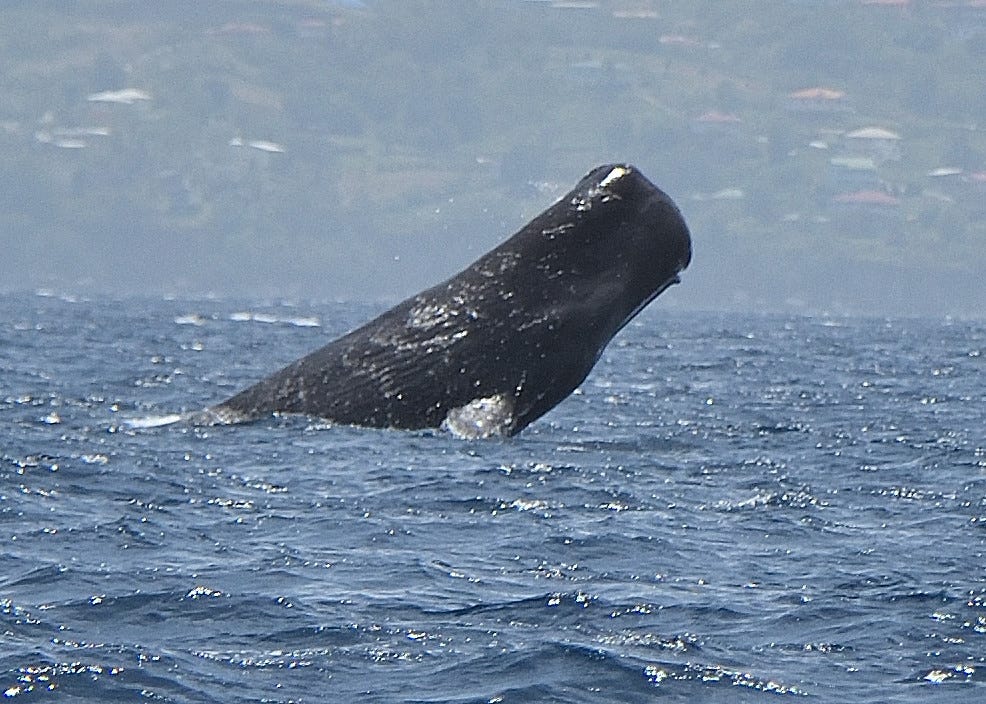The photograph captures a dramatic moment of a dark gray or black whale breaching the ocean surface near a coastline. The whale, likely a gray whale, is leaping out of the calm, slightly choppy blue water with its mouth closed and eyes appearing shut. The image shows the top half of the whale, including its rounded, square-like head and a visible fin on the side. In the background, a lush green island with colorful houses, scattered trees, and grassy hills rises from the misty horizon, adding depth to the serene scene. The calm water, with a few waves and patches of whitecaps, contrasts with the dynamic pose of the breaching whale. The image seems to be taken from a vantage point close to the waterline, possibly from a boat.